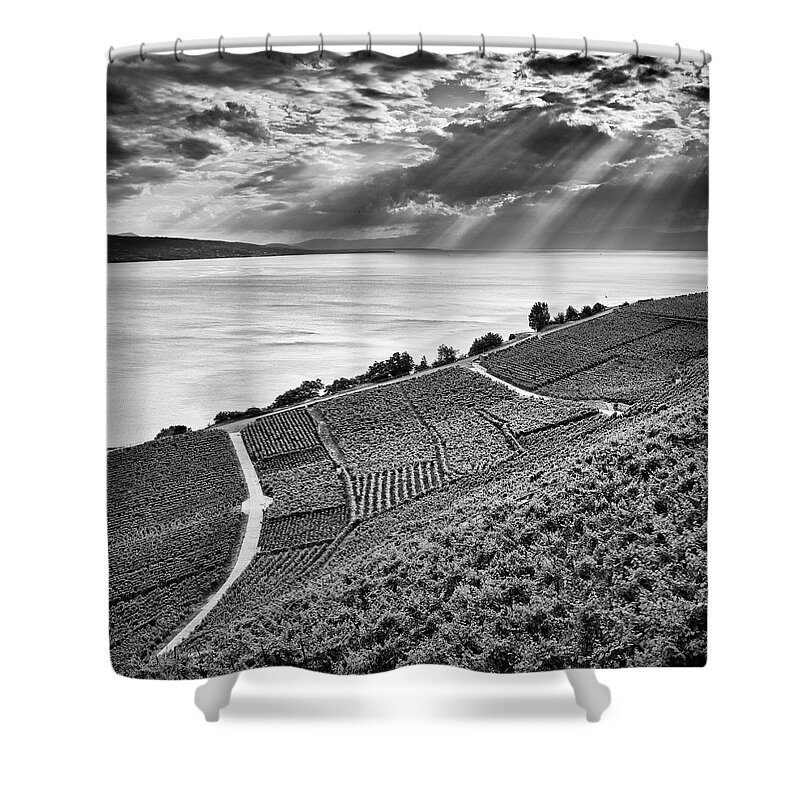This unusual black-and-white photograph is printed on a shower curtain, which hangs from a curved rod with noticeable shower curtain hooks. The image captures a serene, terraced, and landscaped view of agricultural fields leading down to a large body of water, likely a lake, with low hills or mountains in the background. The sky above is dotted with clouds, and striking sun rays beam through, casting light over the scene. The bottom of the curtain has a wavy edge, and the presence of two clawfoot bathtub feet behind it adds an amusing touch, emphasizing that this remarkable image decorates a functional household item.